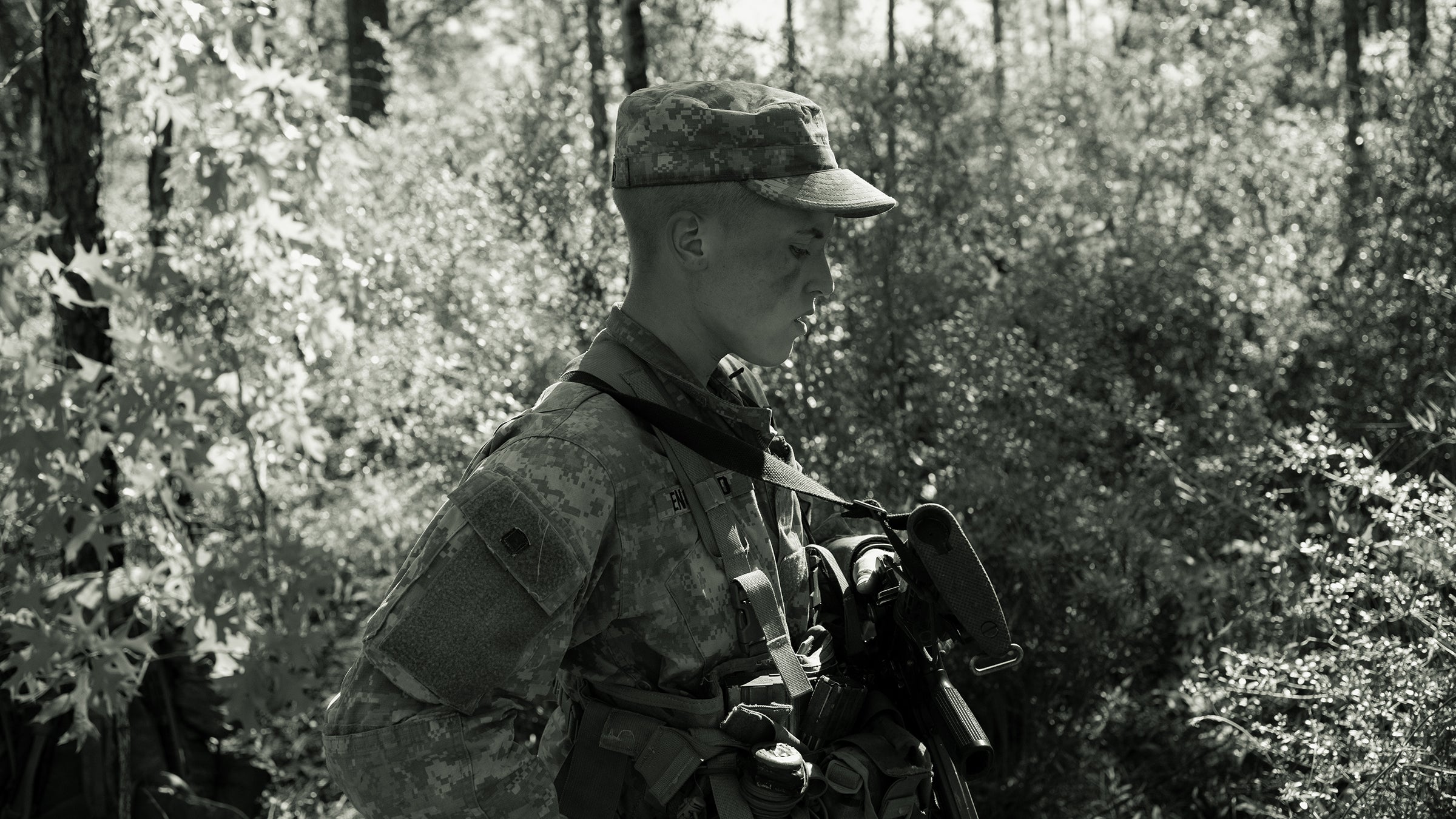The black-and-white photograph depicts a young male army ranger, viewed from the waist up, standing in a forest. He is positioned centrally in the landscape-oriented image, with his body turned to the right and his head slightly bowed as he looks downward. His close-cropped hair is covered by a camouflage cap with a visor. The uniform he wears includes a long sleeve military tunic with velcro sides, uncovering pockets underneath, and a patch pocket with a button closure visible on his upper arm.

Strapped across his chest is a tactical harness made of various nylon straps, holding multiple pouches and possibly grenades. A black nylon strap drapes over his shoulder, connected to a rifle pointed out of frame. A soft beam of sunlight filters through the forest, illuminating some leaves to the left, casting a subdued light on the scene. The overall aesthetic is one of representational realism, meticulously capturing the details and textures in shades of gray, emphasizing a deliberate effort to evoke an aged, historic feel despite the modern setting.